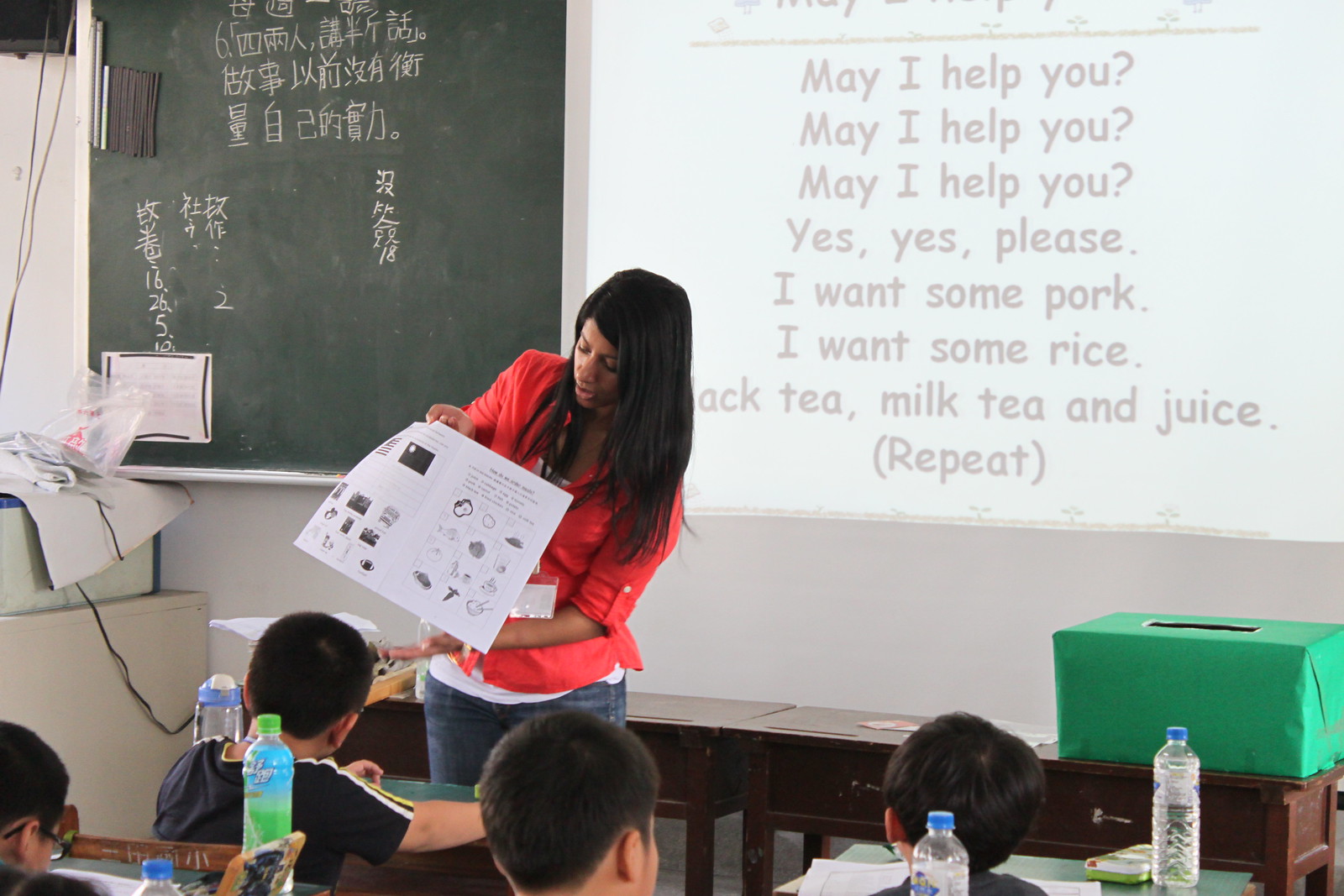In a brightly lit, landscape-oriented color photograph, a classroom scene unfolds with a focus on language learning. Central to the image, a black woman with long dark hair stands at the front of the room, engaged with her students. She wears an orange blouse and blue jeans and holds a white piece of paper, possibly a handout or lesson material, which she appears to be referencing or preparing to distribute. The classroom is populated by four young Asian boys seated at desks in the foreground, each equipped with a water bottle and paper. 

The backdrop of the scene is divided between a chalkboard on the left, featuring foreign language notations in white chalk, and a white projector screen on the right. The projector screen prominently displays a series of English phrases: "May I help you?" repeated three times, followed by responses including "Yes, yes, please," and requests for various items such as "pork," "rice," "black tea," "milk tea," and "juice," with the directive "repeat" at the bottom. A green suggestion box sits on a long brown table beneath the projection screen, adding a pop of color to the otherwise educational setting. This photograph captures a moment rich in detail and cultural interaction, emphasizing the dynamic of an English language lesson in progress.